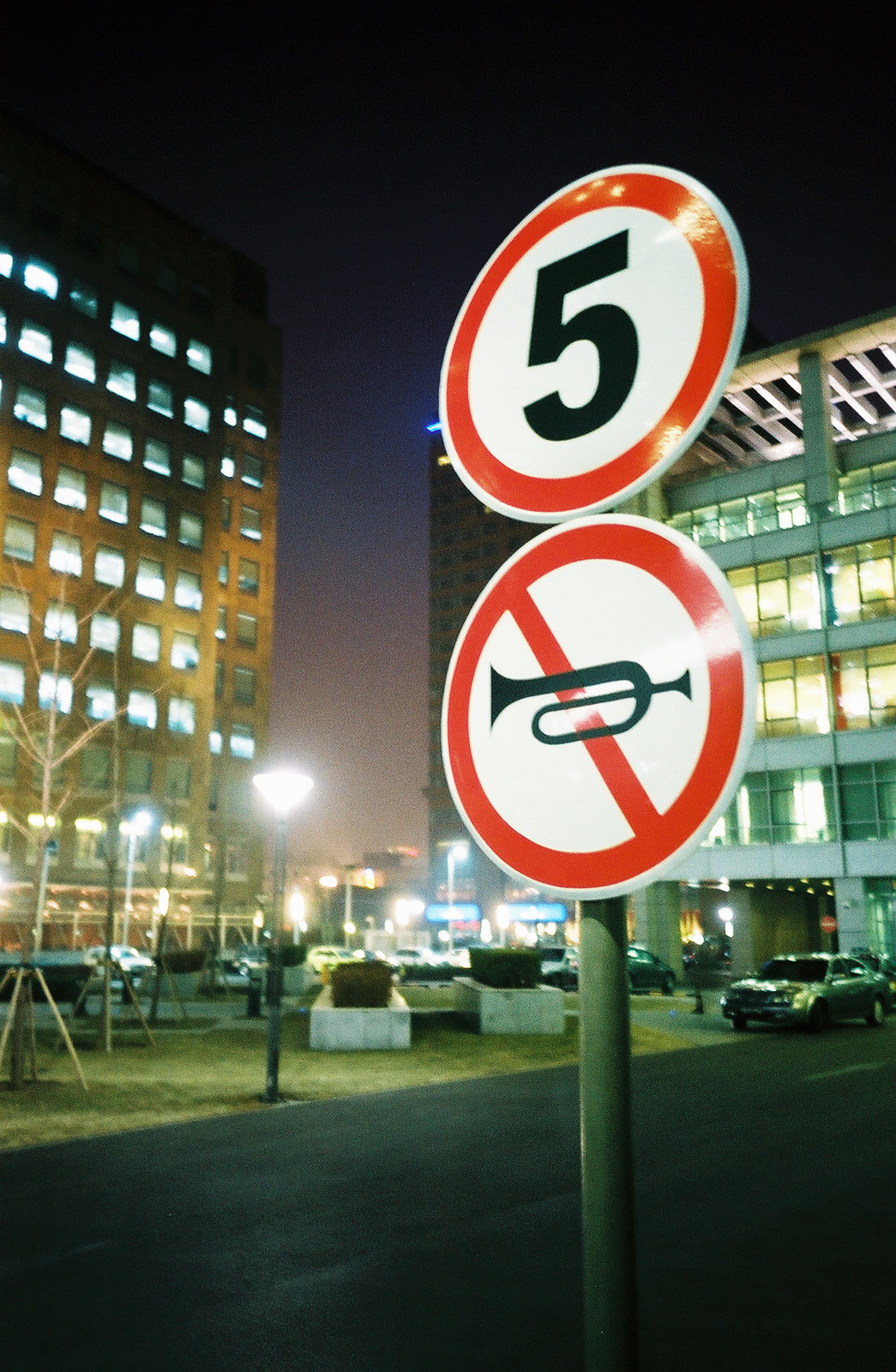In this night-time urban setting, a detailed photograph captures a silver pole with two circular signs, both featuring a white background and red border. The top sign displays a black number "5," while the bottom sign, indicating "no music," showcases a black horn with a slash through it. The scene unfolds in front of multiple buildings bathed in artificial light. On the left, a high-rise building with a light brown facade stretches eight to ten stories high, resembling a waffle due to its square windows. Adjacent is a large, gray, four-story structure, and in the center stands a dark brown building with illuminated storefronts. The setting includes street lights, an outdoor parking area with silver cars, and a small green space with leafless trees supported by wooden braces. The overall scene lacks visible stars and people, emphasizing the city's nocturnal ambiance.